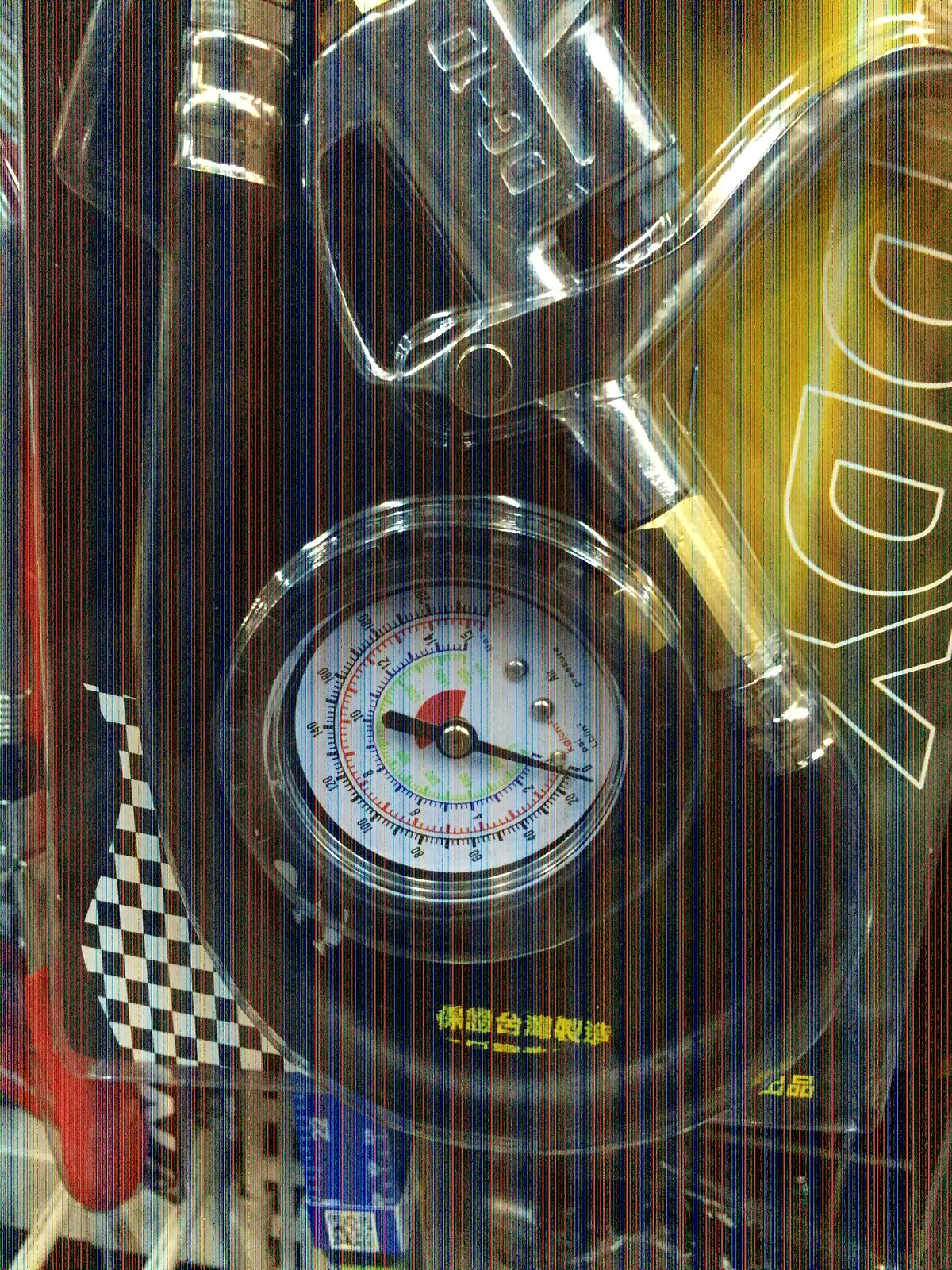An overhead photograph depicts an assortment of automotive-related items against a brown and yellow surface. The image is notably marred by numerous fine blue and red vertical lines, reminiscent of pixel damage on a faulty screen, roughly over 100 lines distributed evenly from top to bottom.

In the lower-left corner, a black and white checkerboard pattern provides a backdrop for a dial situated at the center. The dial, edged in silver, seems to be an air pressure gauge though it bears no identifying labels. The gauge features two numbered scales: an outer circle ranging from 0 to 75 and an inner circle from 0 to 15, traversed by a black pointer.

Adjacent to this gauge, towards the middle right, lies an object resembling a miniature gas pump nozzle with a stainless steel handle. Engraved on the handle are the characters "DD-10." Additionally, to the far right, yellow and brown letters outlined in white spell out "DDY," completing the compilation of car-related items in this image.